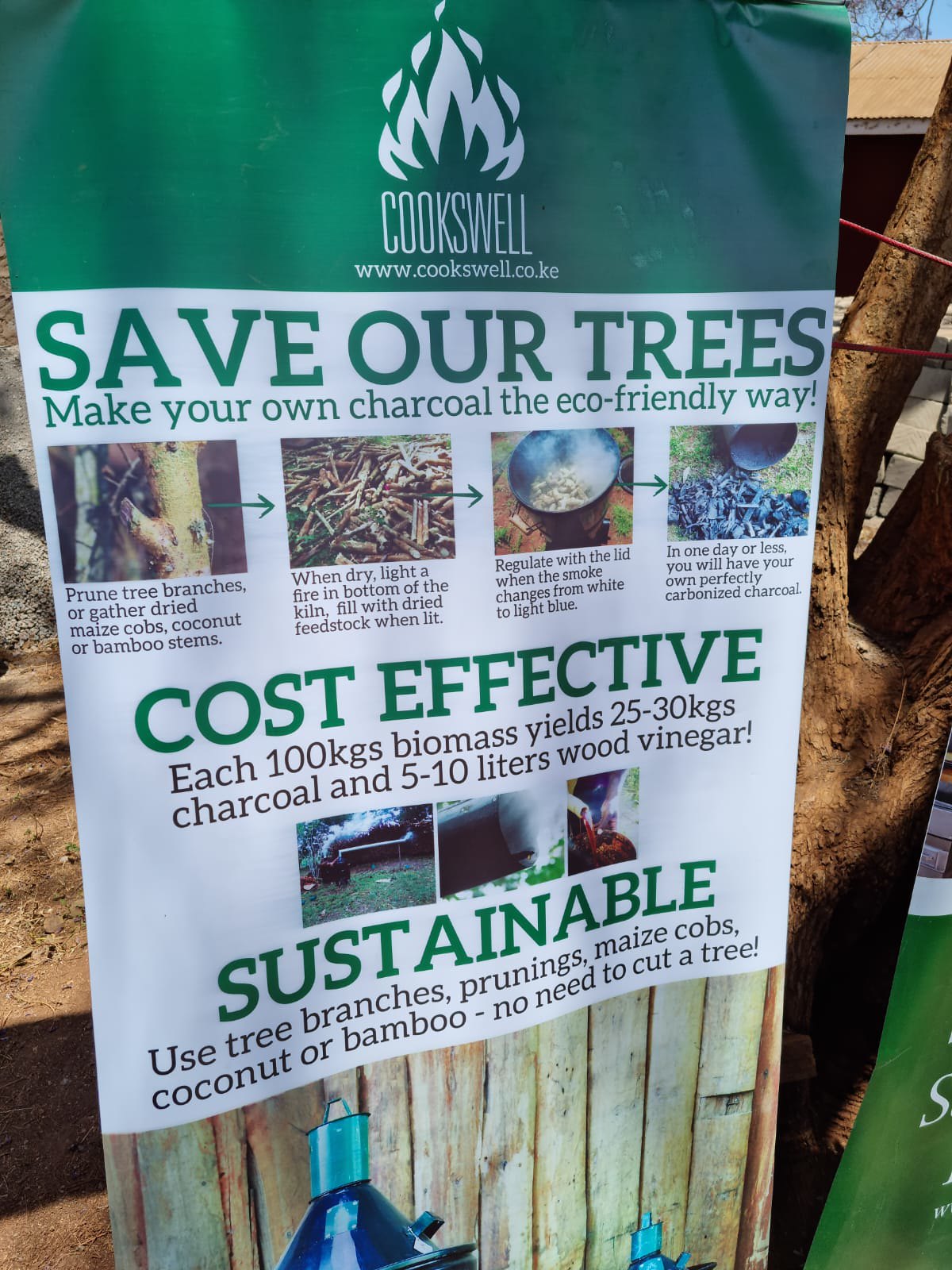The image features a large, thin vinyl banner suspended, likely from a tree, as evidenced by a prominent tree branch on the right side of the image. The banner's design is divided into sections, primarily green and white, with detailed eco-friendly information. At the top, a green section displays the Cookswell logo alongside the web address "www.cookswell.co.ke". Beneath this, in a large green font on a white background, the banner proclaims "Save Our Trees". It details a step-by-step process for making eco-friendly charcoal, advising to prune tree branches or gather dried maize, cobs, coconut, or bamboo stems. Instructions include lighting a fire in a kiln with dried feedstock and regulating it until the smoke changes from white to light blue, yielding perfectly carbonized charcoal in a day or less. Additional text highlights that each 100 kilograms of biomass produces 25 to 30 kilograms of charcoal and 5 to 10 liters of wood vinegar, emphasizing cost-effectiveness and sustainability. The lower sections of the banner feature photographs and further instructions on producing charcoal and sustainability tips. The bottom of the banner partially shows a picture with a wood fence and some bottles, presumably the end product or part of the process.